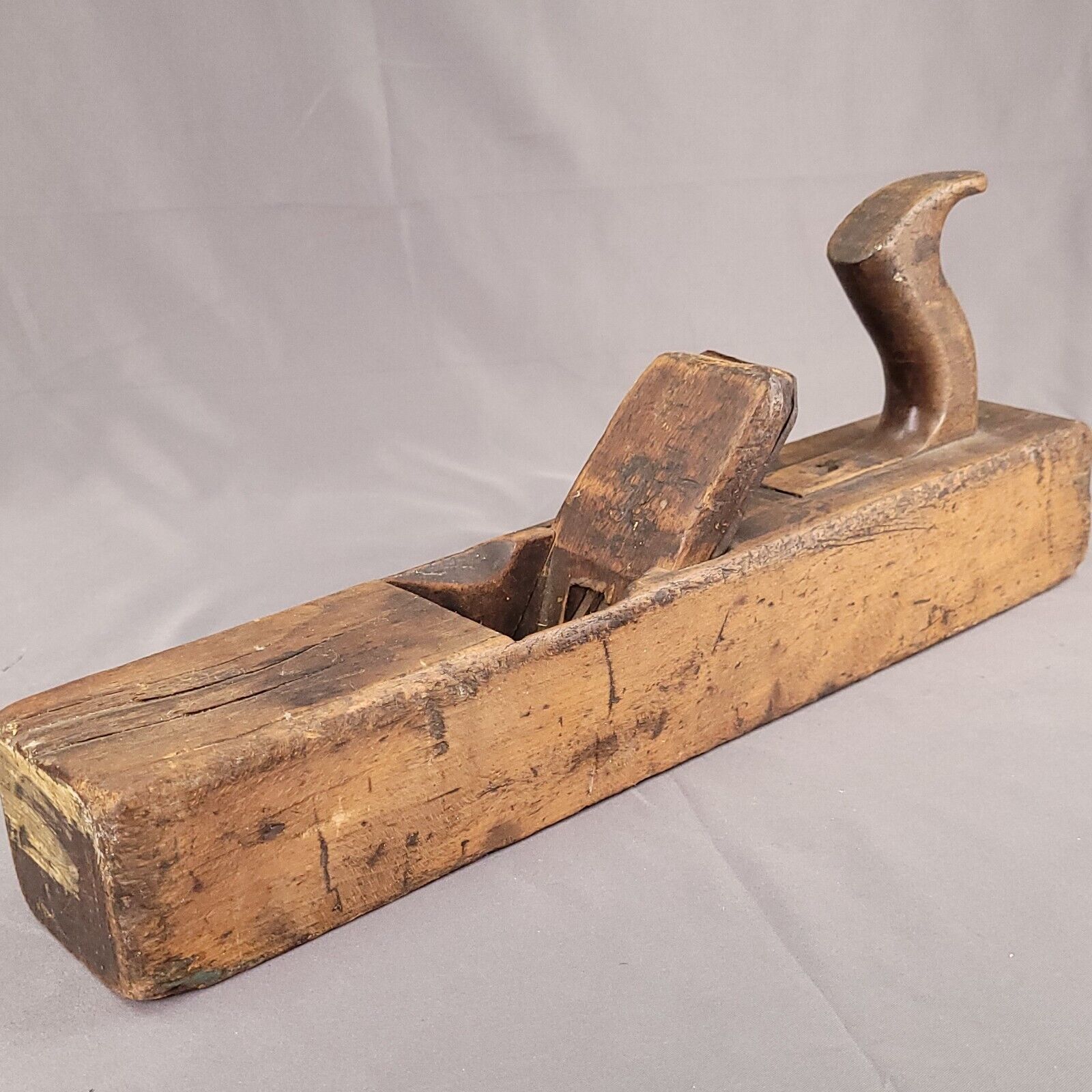In the image is an antique, rectangular wooden device, likely a tool, placed on a flat surface covered with a white or possibly slightly purple cloth. The wood, exhibiting significant wear, stains, and cracks indicative of its age and potential humidity damage, is thick and weathered. The object features a square hole in the middle with a wooden lever or button protruding from it. On one end of the device is a large, curved wooden handle, resembling a bird’s neck and head, arching upwards. Despite its age, the tool remains in relatively good condition, capturing a glimpse of craftsmanship from the olden days.